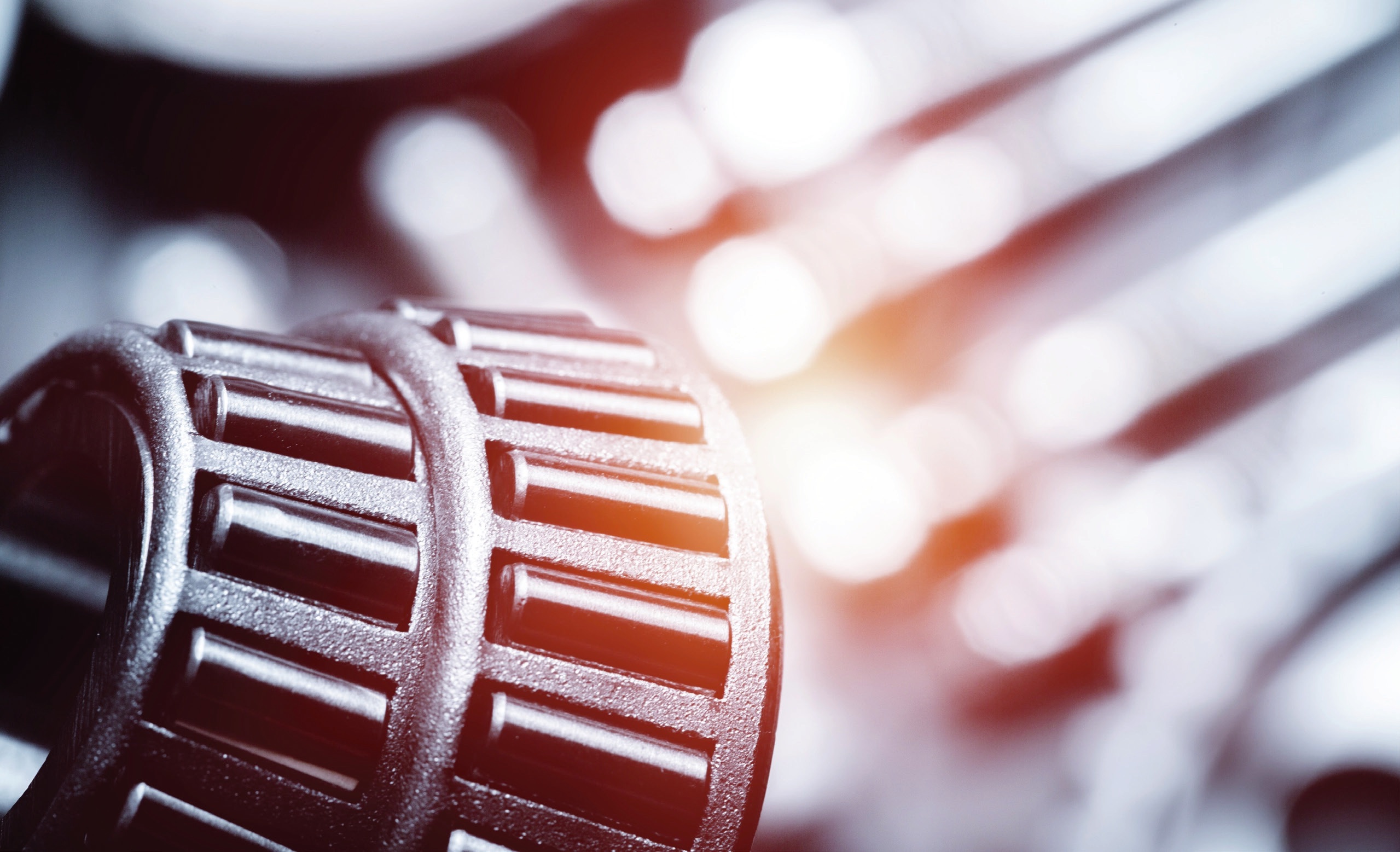The image features a metallic object on its side positioned in the lower left-hand corner of the photo. This object resembles a bucket or possibly a microphone, characterized by line patterns and a series of circular, stacked rings, with the bottom ring being thicker than the top. The metal surface appears silvery-white and somewhat shimmery. To the right, the image fades into a blur dominated by bright, streaming light with white and slightly orange glares, giving an overexposed appearance. The background is out of focus and contains dark areas at the top and left sections, with the right side featuring projections that extend diagonally, resembling tubes with rounded ends.